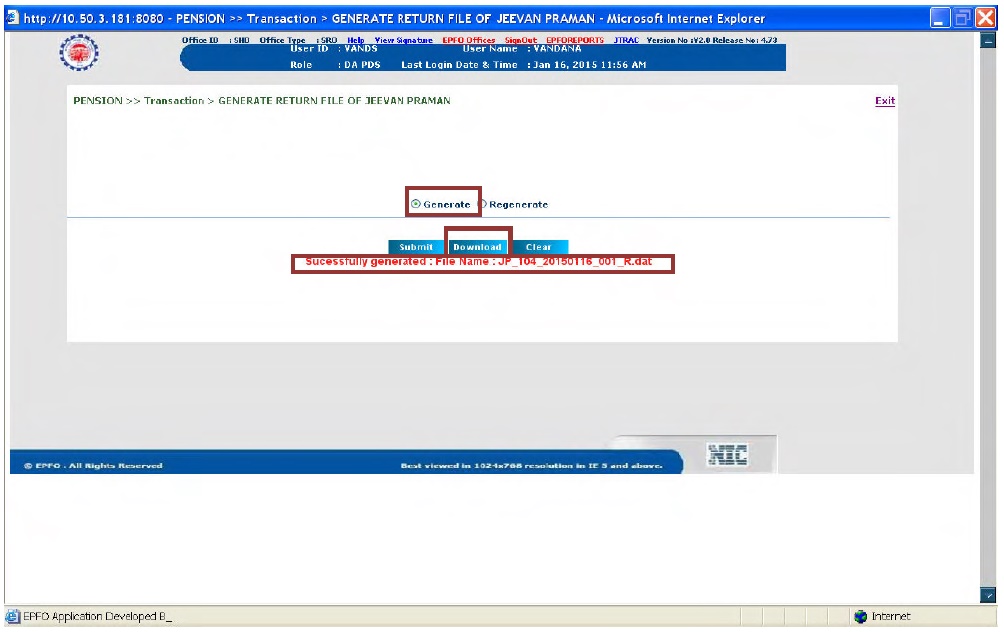The image depicts an Internet Explorer window with a visible URL and various interface elements. At the top, there is a blue rectangular bar which contains the URL "http://10.50.3.181:8080-pension >> Transaction >> Generate a return file of GVanPraman - Microsoft Internet Explorer," written in white text. Below this bar is a light gray background displaying user information including username, role, and last login date and time, all formatted in white text. This information is enclosed within a dark blue, rounded rectangular border on the left side.

Further down, there is a large white rectangular section featuring options highlighted in green text. Some of these options, specifically "generate," "download," and "successfully generated: file name (with the file name provided)," are outlined in red to emphasize their importance. Below this, the predominant background remains light gray, providing a neutral backdrop for the rest of the interface elements.